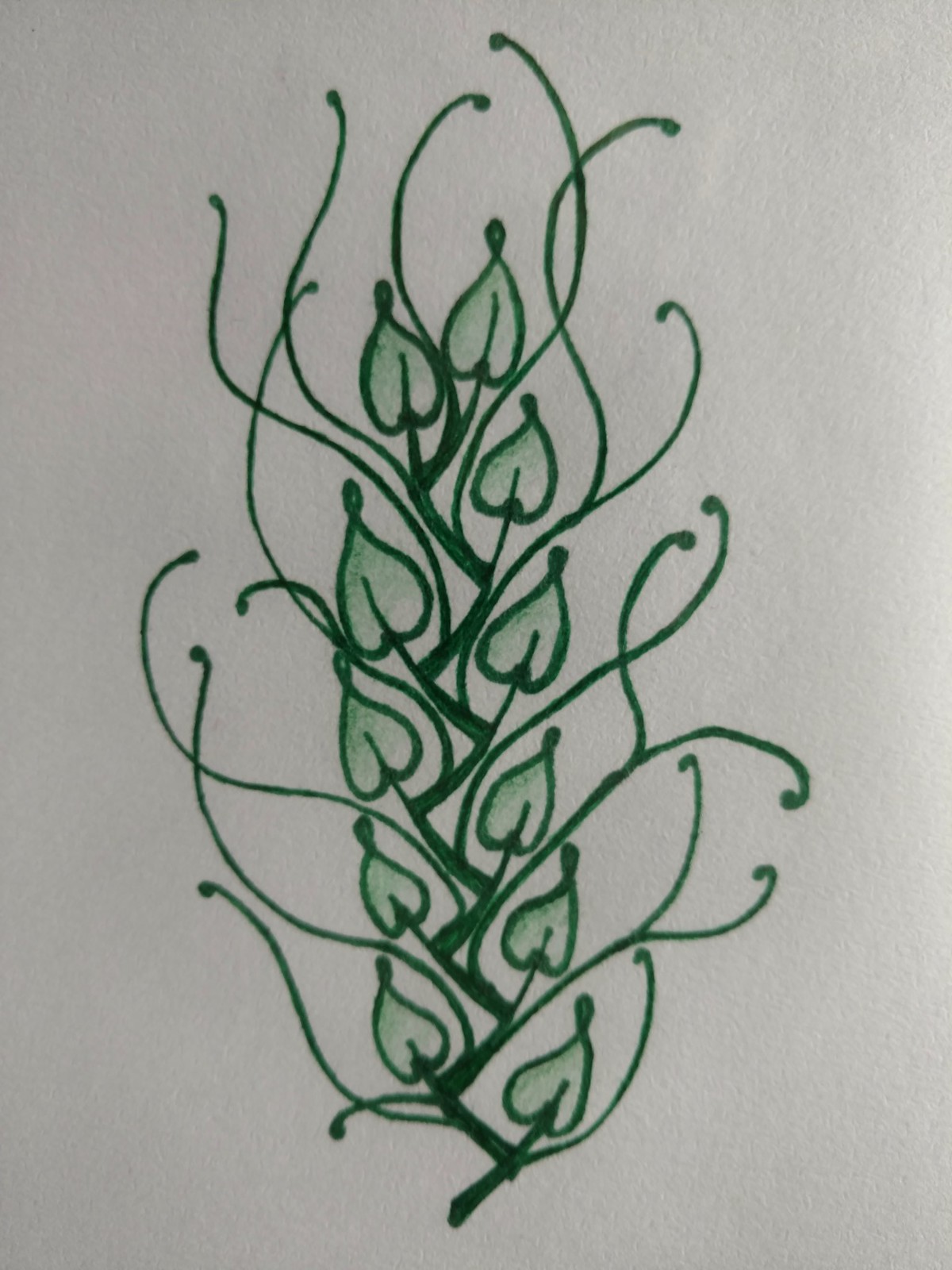This photograph captures a close-up of a person's detailed drawing on white paper. The artwork features a central, thick green zigzag stem, meticulously rendered with a marker. From this main stem, several spear-shaped, heart-like leaves branch off, each outlined in green and filled in with lighter green colored pencil or crayon. The leaves, resembling inverted hearts with central veins, present a dynamic texture. Extending from these leaves are delicate, curly vines, each terminating in a soft curl. The overall impression is reminiscent of a climbing vine in motion, though the realistic depiction of nature intertwines with an almost decorative, artificial plant aesthetic. The off-white, textured background of the paper enhances the drawing's intricate details, highlighting the play of light and shadow across the overlapping leaves and twisting tendrils.